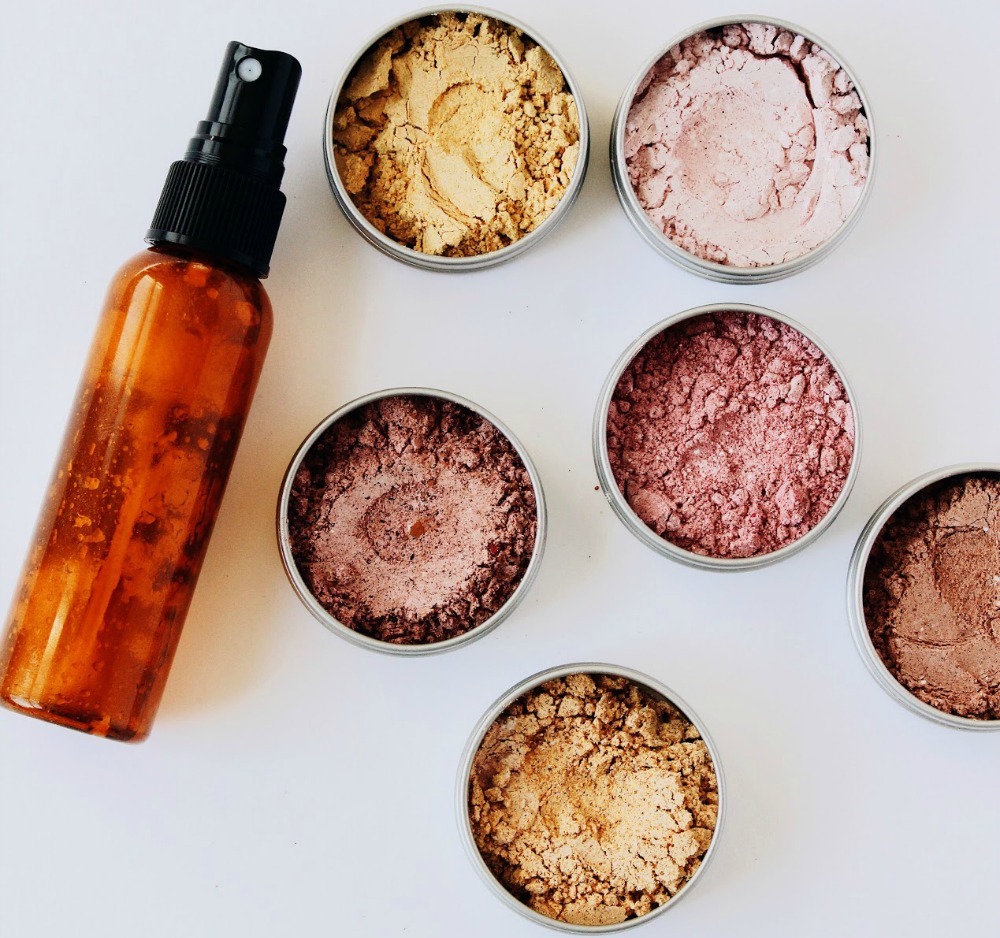An overhead photograph captures six silver tins filled with variously colored powders, likely cosmetic makeup, arranged on a white table. The tin colors from top to bottom include gold, light pink, dark brown-red, pink-dark red, golden brown, and a cropped dark brown tin on the right edge of the image. Each tin is distinctly visible with a different shade of makeup powder, contributing to a visually rich array. Positioned to the left of the tins is a small, see-through spray bottle containing an orange or amber fluid, topped with a black cap and spray nozzle directed towards the viewer. The setup is illuminated by a light source from the left, casting a noticeable shadow from the spray bottle, further defined against the white backdrop.